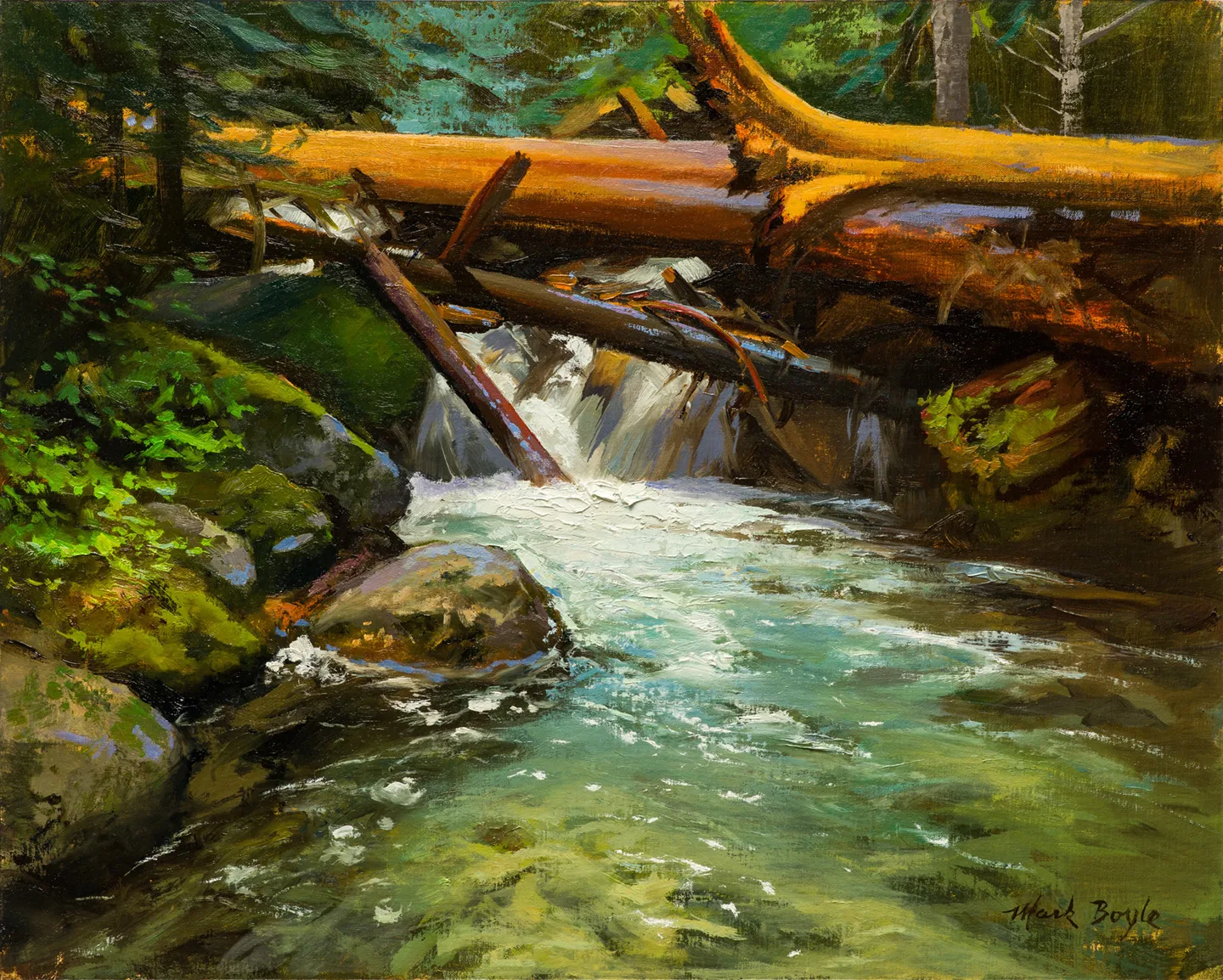The painting, possibly an oil piece done in a wet-on-wet style, depicts a detailed and photorealistic forest landscape surrounding a small stream. The stream flows diagonally from the bottom left, bubbling through rocks covered with moss and grass. The rocks and bank on the left are adorned with green vegetation. In the middle of the painting, slightly towards the top, fallen tree trunks—some light brown and thick—sprawl across and into the water, creating a series of small waterfalls. The trunks appear tangled and layered, contributing to the dynamic flow of the stream. Above the waterfalls, the backdrop features a mix of pine trees and a serene gradient of green and blue hues, adding depth to the forest scene. Notably, the artist's signature is visible in the bottom right corner, reading "Mark Boyle," confirming the creator's identity.